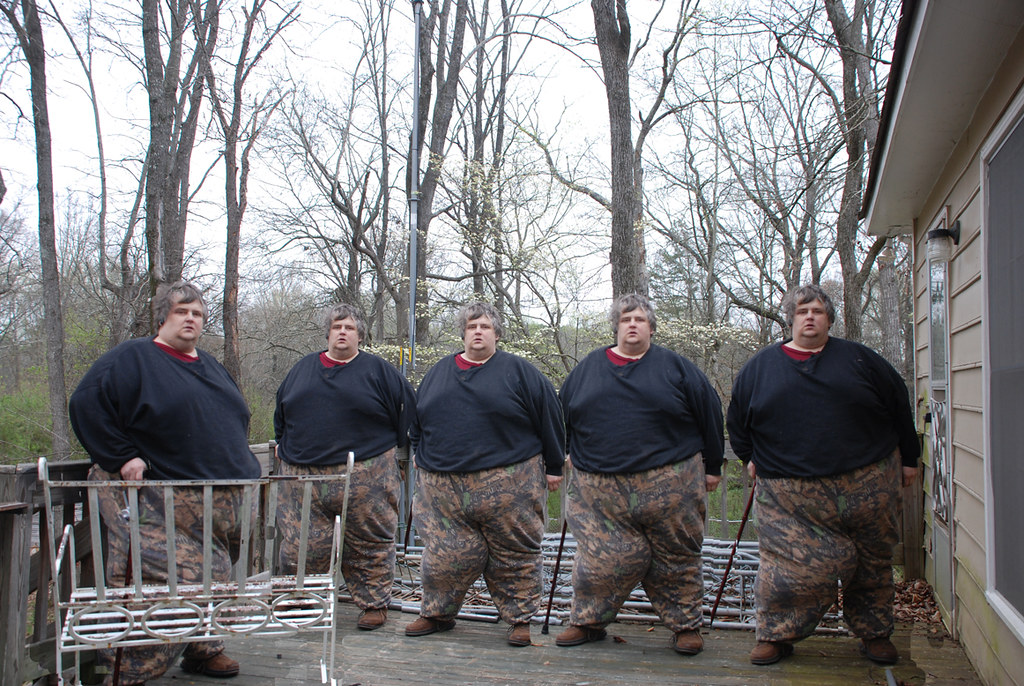In the photograph, an elderly, obese person with salt-and-pepper hair appears five times, creating the illusion of duplicates. They are standing on a weathered gray wooden deck, which is part of a house with a cream color and white trim around the windows. The person is dressed in long-sleeved black or dark blue shirts over a red undershirt, camouflage pants, and brown shoes. Four of the images show the person standing front-facing, side by side, while the fifth shows them turned sideways. The individual uses a cane, hinting at mobility issues. Their expression is monotone, neutrally staring into the distance.

The deck also features an aged white metal rocking bench, along with other metal railings. The backdrop includes a wooded area, likely in early spring, as the trees are bare but starting to bud. The photo, taken during the day, captures the vastness of several large brown trees extending horizontally across the top portion of the image. Additionally, parts of the house, including a light, door, and window, are visible on the right side of the frame.